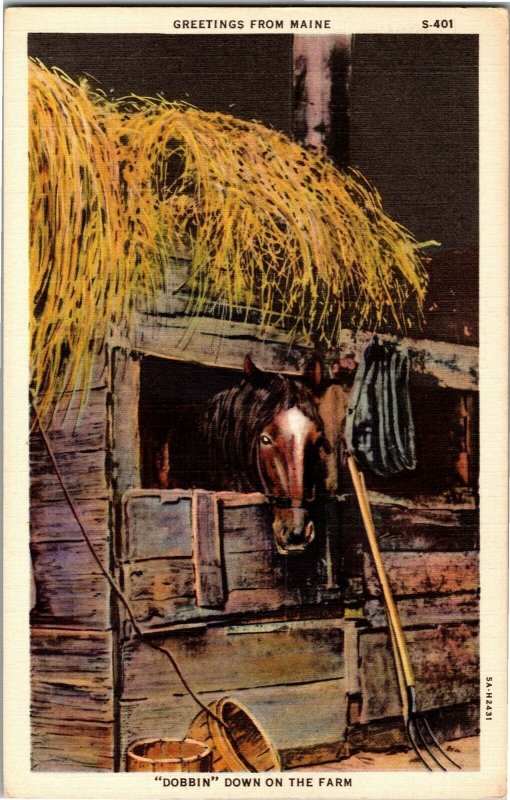The image is an old-fashioned postcard, yellowed with age, featuring the caption "Greetings from Maine" at the top and "Dobbin, down on the farm" at the bottom. The main image appears to be a hand-colored photograph or painting of a rustic, makeshift stable constructed from scrap wood. Poking its head through a small window in the stable is a beautiful brown horse named Dobbin, with a black mane and perked-up ears, gazing directly at the viewer. Leaning against the stable wall is a large pitchfork, and the ground in front is adorned with two wooden buckets or barrels. Above the stable door, long strands of hay hang down, suggesting storage overhead. Additionally, a halter or harness dangles beside the door. The postcard is identified with an image number "S-401" in the upper right corner.